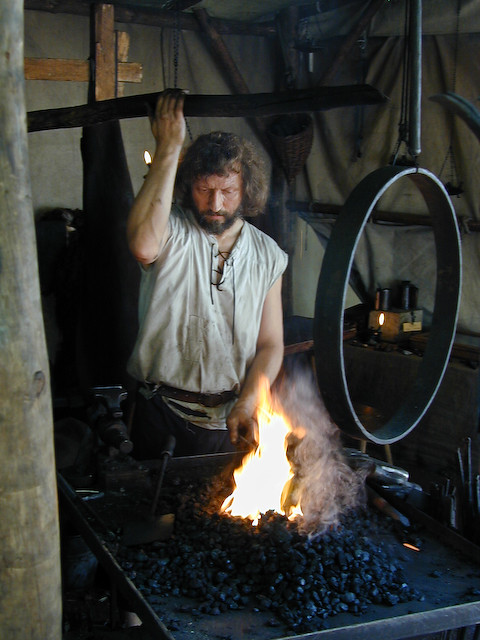In the image, a man who appears to be a blacksmith is captured in his workshop, which resembles an old-fashioned stall or tent with canvas walls and wooden beams. The man, likely in his 40s, has long, somewhat unkempt brown hair and a matching beard and mustache. He is a white man dressed in a Renaissance-style, white short-sleeve shirt with laces instead of buttons on the front, tied loosely. His left hand reaches out towards a fire erupting from a bed of coal on a cast-iron table or pit, while his right hand grasps a wooden beam just above his head for support. Above the fire pit, to the right, hangs a large metal ring from the ceiling. The intensity of the fire contrasts with the otherwise dimly lit, smoke-filled environment, adding a sense of focus and urgency to the blacksmith's work.